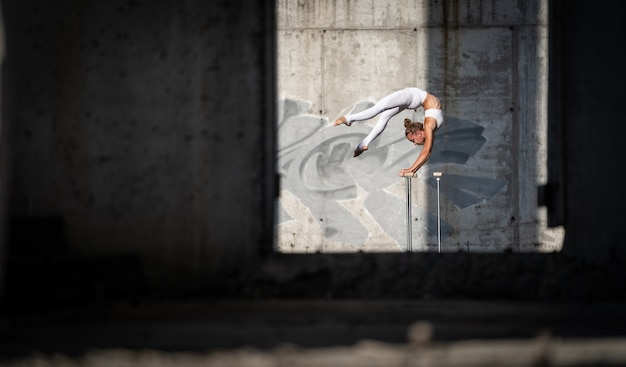The professionally taken full-color photograph captures a gymnast performing an impressive handstand on a balance beam in a horizontally rectangular frame. The gymnast, illuminated by focused lighting within a square area, wears white leotards and a matching white sports bra. Her hair is neatly tied up in a bun. She balances on her hands with her legs elegantly arched over her head, bringing her feet nearly level with her hands. This athletic pose highlights her strength and flexibility. The background features an older-looking stone wall with large rectangular sections, adorned with a gray flower artwork. Two metal poles supporting the horizontal balance beam are visible, and the lady is grasping the bar mid-routine. The rest of the image subtly fades into a dark grayish-black shade with a speckled stone-like texture, creating a stark contrast that draws the viewer's focus onto the gymnast's incredible performance.